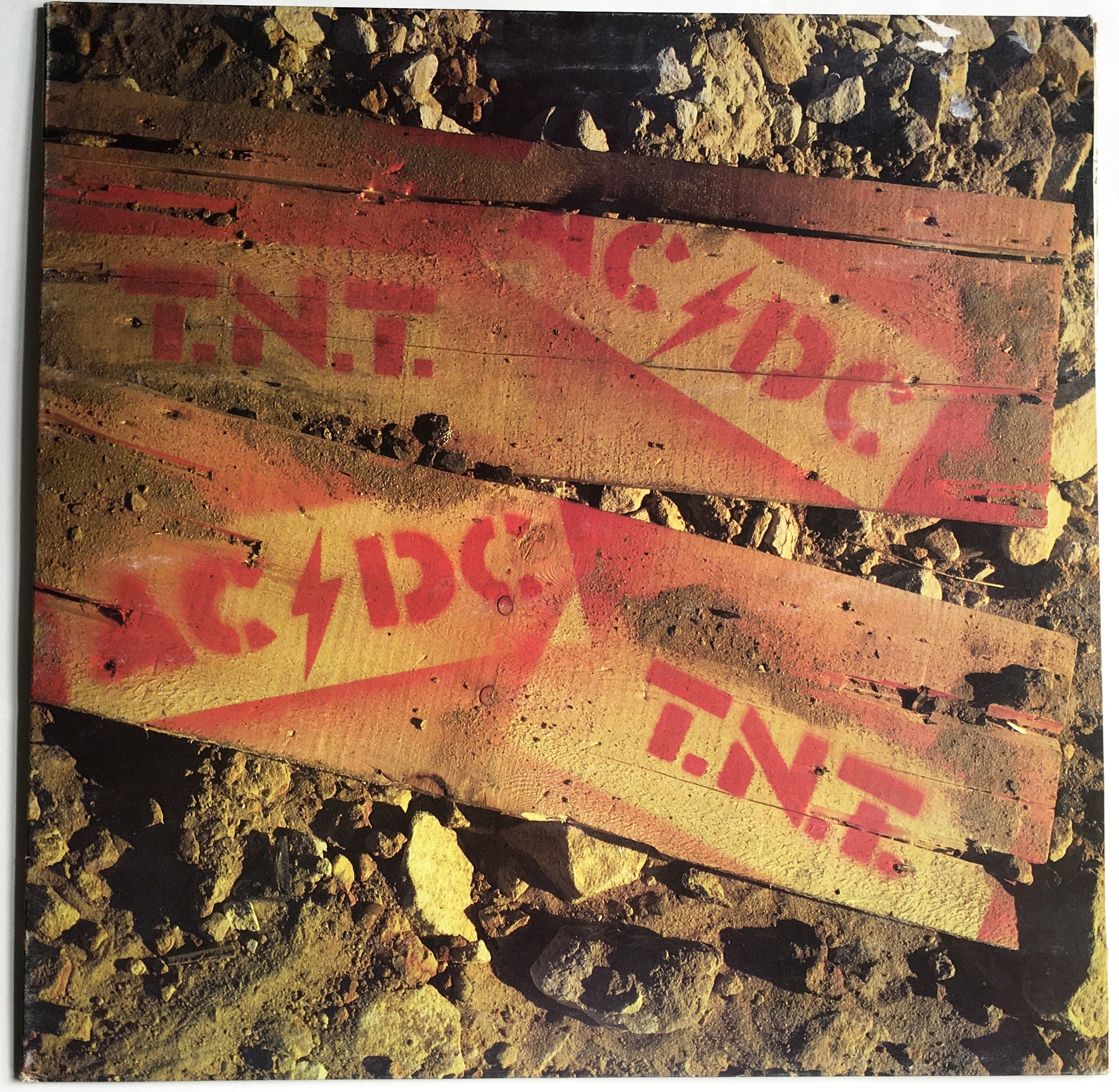The image features two weathered, rectangular wooden boards laid on a rocky terrain, angled slightly to each other. The boards are predominantly a reddish-brown color, but the sections where logos are spray-painted are lighter. The top board displays "TNT" in bright red on the left side, while the bottom board features "ACDC" in the middle, divided by a red lightning bolt, and these inscriptions appear repeated in a scattered manner. The background is filled with dark and light gray rocks, with minor patches of gray dirt towards the lower part. The setting is outdoors, captured in a close-up that focuses on the distressed wooden boards and the rocky ground, emphasizing a scene that evokes themes of ruggedness and decay, possibly inspired by the song "TNT."